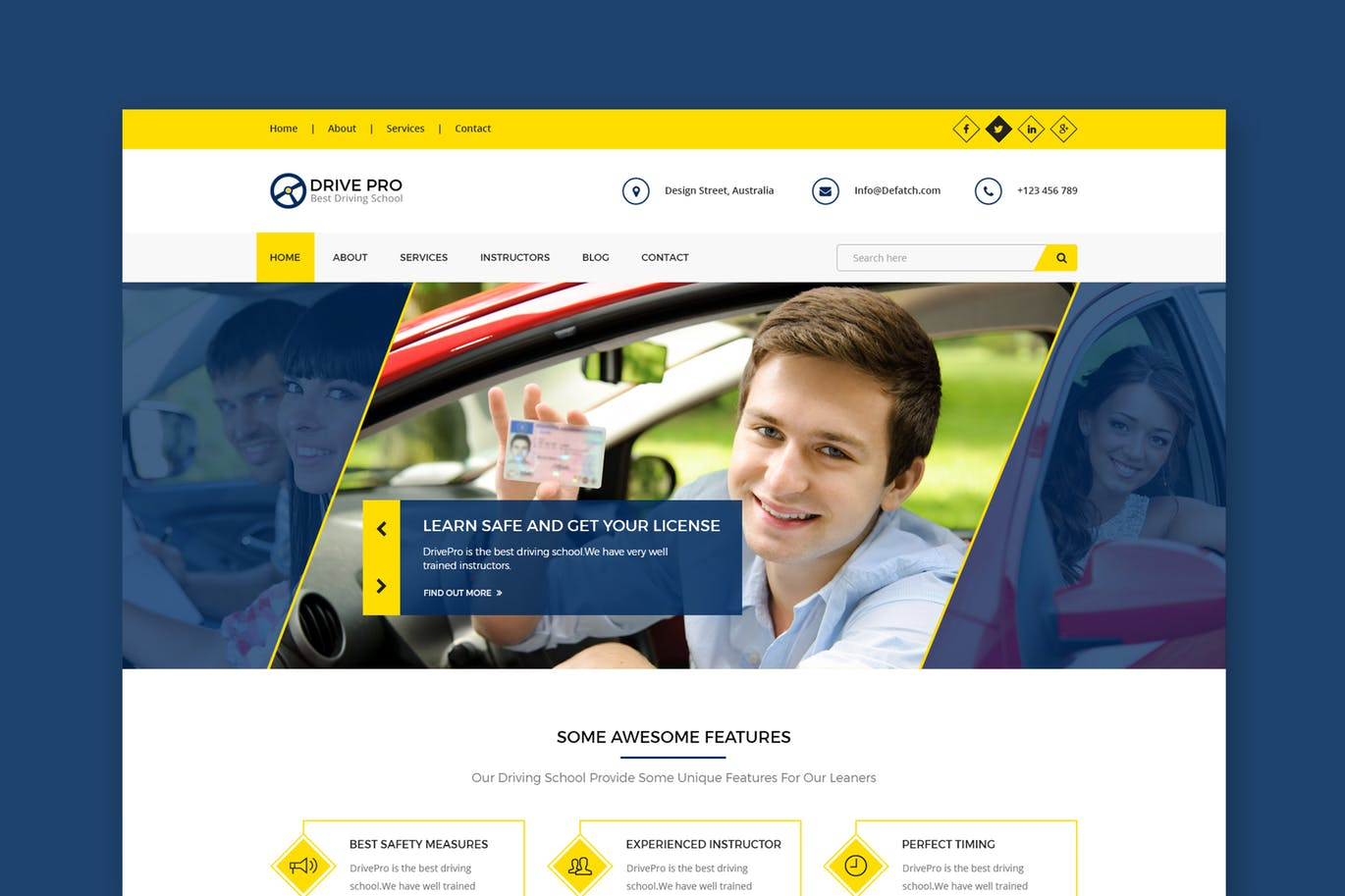The web page features a navy blue border with a prominent yellow banner running horizontally across the top. The banner displays the navigation menu in black text, listing: Home, About, Services, and Contact. On the right side of the banner, there are four outlined icons for social media platforms—Facebook, Twitter, LinkedIn, and Google Plus.

Below the banner, the main section of the page has a white background. To the left, the header reads "Drive Pro" followed by a subheading "Best Driving School" accompanied by a small navy steering wheel icon. To the right, there is a contact section labeled "Design Street, Australia," which includes an email address (info@defetch.com) and a phone number. Next to the Design Street label are icons within blue outlined circles: a location icon, an envelope, and a phone.

Beneath the header, there is a secondary navigation menu in black text listing: Home, About, Services, Instructors, Blog, and Contact. The "Home" link is highlighted inside a yellow box. Adjacent to this menu on the right side is a search bar labeled "Search Here."

The central image depicts a young man, likely a high school student, seated in a car and proudly holding up his driver's license. Below this image, a banner is displayed, with a message that reads "Learn Safe and Get Your License" on a navy blue and yellow background, followed by "Drive Pro is the best driving school," and an arrow pointing left. There is also a "Find Out More" prompt with an arrow pointing right.

At the bottom middle of the page, against a white background, a section titled "Some Awesome Features" highlights unique offerings of the driving school. This section is divided into three parts, each outlined in yellow:
1. "Best Safety Measures" - Partial text: "Drive Pro is the best driving school we have, well trained…" (cut off)
2. "Experienced Instructor" - Partial text: "Drive Pro is the best driving school we have, well trained…" (cut off)
3. "Perfect Timing" - Partial text: "Drive Pro is the best driving school we have, well trained…" (cut off)